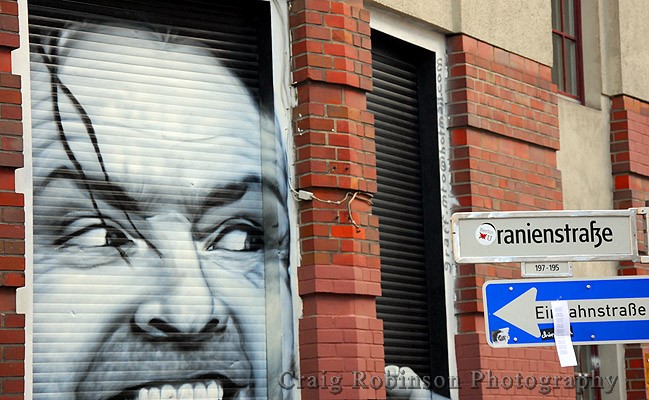The image depicts the exterior of a city building. The bottom section of the building is constructed out of red bricks, while the upper parts feature lighter tan bricks and cement panels. On the left side, there's a garage door with a white frame, and on the door, there's a black and white art piece of Jack Nicholson's face from the movie "The Shining," where he has a crazy expression. To the right of the art, on the building wall, two street signs are visible. The top sign is a white rectangle with black text "R-A-N-I-E-N-S-T-R-A-F 3" and some unreadable small white circles with a little red symbol. Below it, there's a blue street sign with a white arrow pointing left. The text is partially obscured by a receipt, reading "E-I-A-H-N-S-T-R-A-B-E."